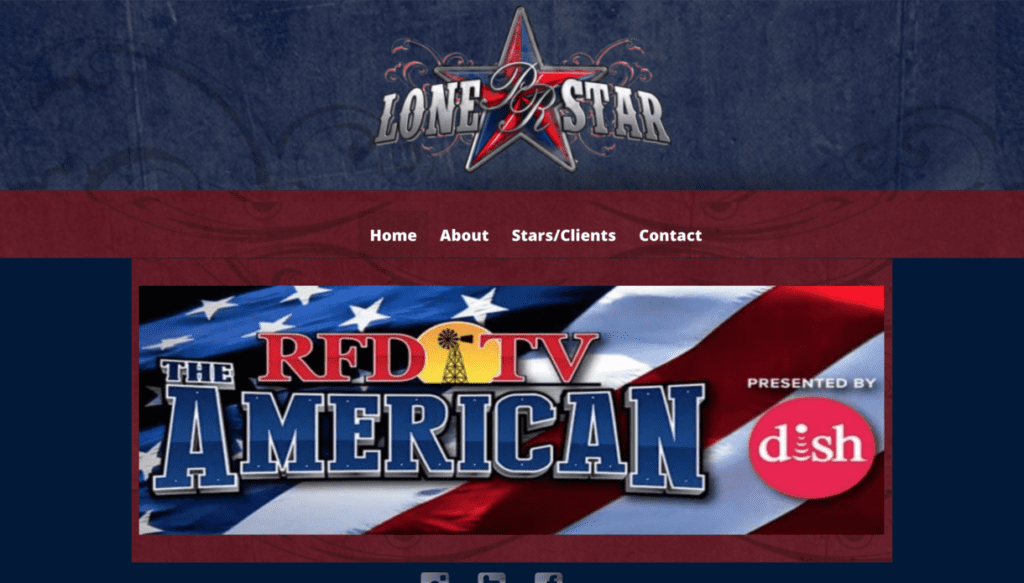The image is a rectangular screenshot, likely from a website or an ad for a TV show, called "LoanStar." The primary color of the site is dark blue, with an old-fashioned paisley pattern decorating the top bar. At the top center, "LoanStar" is displayed over a red and blue star. Below this, a thinner maroon band spans horizontally across the page, containing white text that reads "Home, About, Stars, Clients, and Contact."

The webpage prominently features a banner in the center. This banner includes a patriotic-themed design with an American flag background. Over the flag, large red text reads "RFD TV American," with "RFD" and "TV" in red and "American" in bright blue outlined in white. Between "RFD" and "TV," there is a yellow sun containing a black windmill. Above this text, in smaller white letters, it says "presented by," referring to Dish Network, which is indicated by a red circle with "dish" written in white within it.

The overall layout and design give a distinctly patriotic and classic American aesthetic.